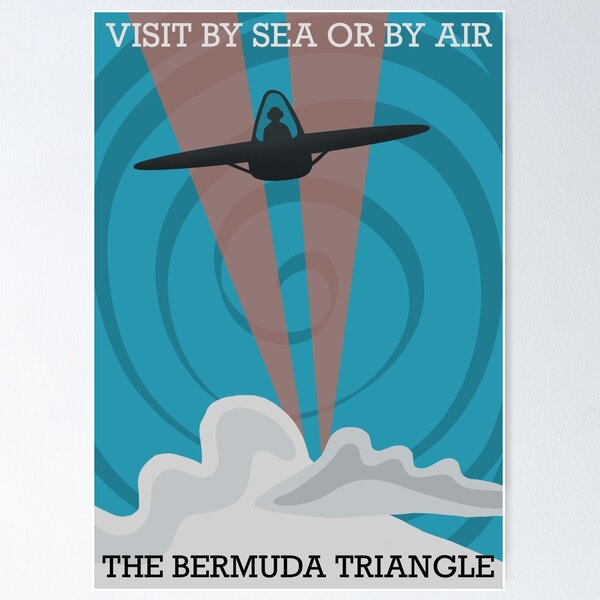The image features a square poster, approximately 4 inches by 4 inches, set against a light gray background. The poster itself is rectangular, slightly smaller than the square background, with a thin white pinstripe outline. It has a blue background centered by a dark blue spiral that expands outward, accompanied by a lighter blue swirl. At the top, in bold white capital letters, the poster reads, "VISIT BY SEA OR BY AIR." At the bottom, large black capital letters state, "THE BERMUDA TRIANGLE."

Prominently displayed is a silhouette of a single-engine airplane with a visible pilot, depicted in black and flying upward. The plane is set against the blue background. Below, there are white and gray clouds at the bottom of the image, along with two vertical, reddish-brown light beams that widen as they rise from the bottom up. The overall effect suggests a mystical and intriguing representation of travel, emphasizing the enigmatic allure of the Bermuda Triangle.